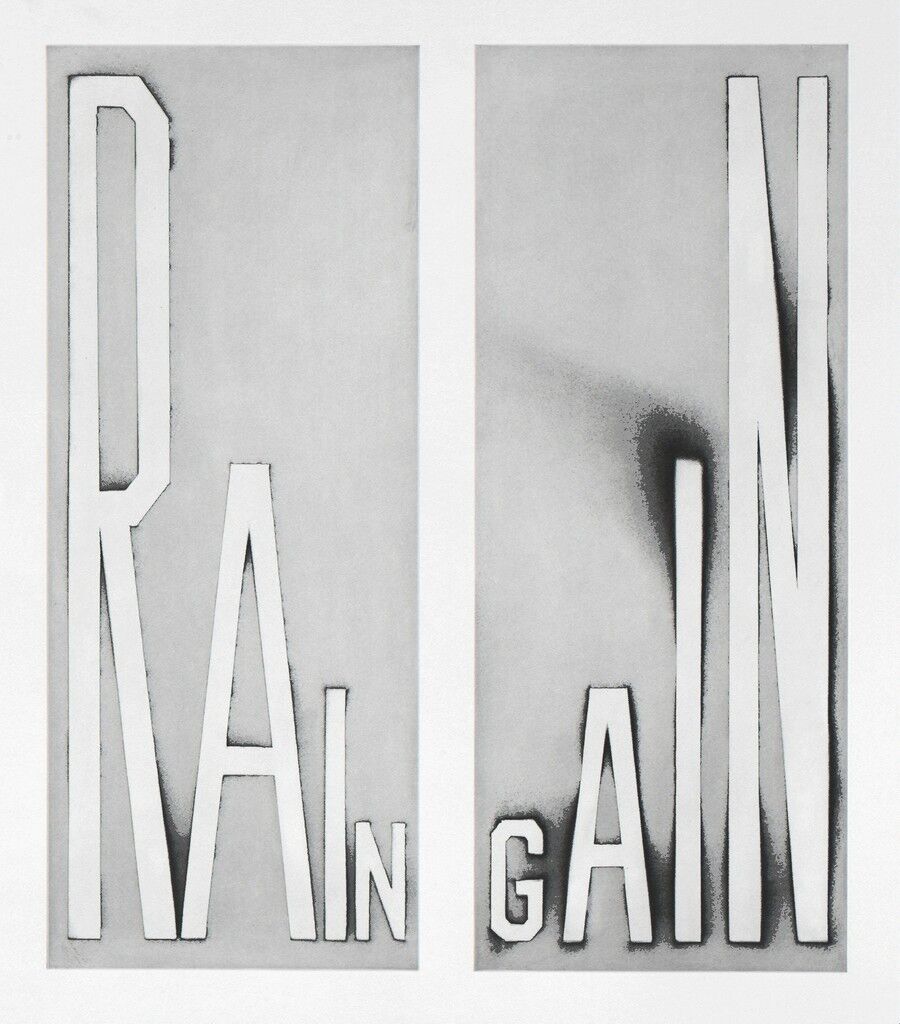The image features a sophisticated and artistic black-and-white poster with a light grey edge framing two tall, vertically aligned rectangular sections that are separated. Each section has a darker grey background. The left section displays the word "RING" in white capital letters, with the "R" being the largest and the letter size gradually decreasing to the smallest "N." The right section features the word "GAIN," also in capital letters but with sizes increasing from the smallest "G" to the largest "N." Both words have subtle shadows behind them, adding depth to the design. The varying font sizes create a dynamic visual effect, lending an intriguing and professional aesthetic that may be promoting an entity or concept called "rain gain" or "rain game" in a distinctive manner.